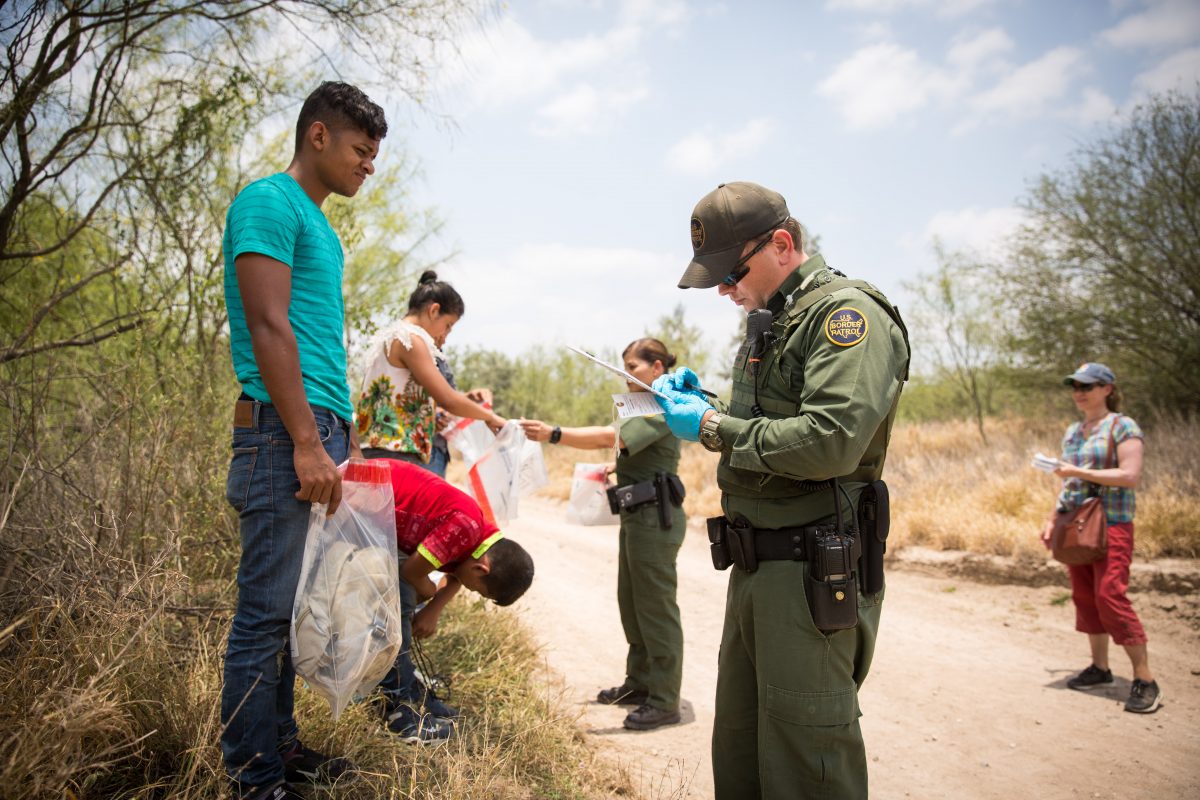In this detailed image, two Border Patrol agents are positioned along the edge of a dirt road, framed by a backdrop of trees and wild growth. The sky above is notably blue with scattered white clouds, casting a predominantly cloudy ambiance. The closer agent, a male with a brown ball cap, sunglasses, and blue gloves, wears a green uniform with a blue and yellow patrol patch on his left shoulder, and his belt is equipped with various accessories, including a walkie-talkie. The other agent, a female without a hat but sporting a black wristwatch, engages with a group of individuals, appearing to be immigrants, who are standing partially in the foliage. This female agent seems to be handing or receiving a bag from a woman in white floral-patterned capri pants, tennis shoes, and carrying a purse.

Among the group of immigrants, two younger individuals stand out; one in a red shirt and blue jeans, another in a blue striped shirt with blue jeans. Others are observed carrying personal items in plastic bags, with one person actively tying their shoe and another managing their belongings. Further back, a civilian woman with a tie-dye shirt, red pants, a blue hat, and black shoes is seen. The dirt road is bordered by brown grass and dense brush, emphasizing the rural setting of this encounter.